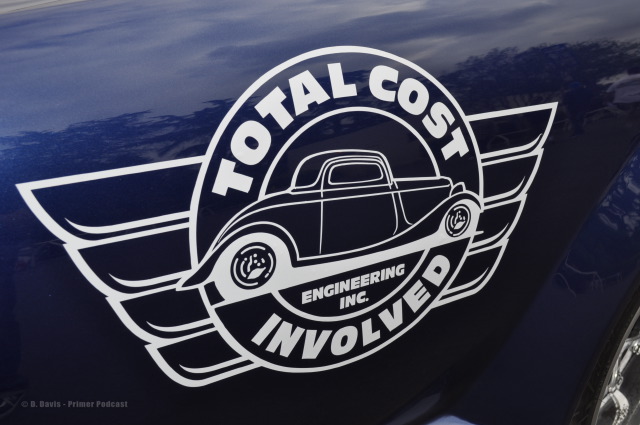The image captures the side of a navy blue, vintage car, glistening as it reflects the surrounding trees, sky, and clouds. Dominating the image is a large white decal, centrally placed on the vehicle's side panel. This decal features a round emblem with the bold text "TOTAL COST" arcing along the top, and "INVOLVED" curving along the bottom. At the heart of the circle is a detailed illustration of a classic, two-seater vintage car, with "Engineering INC" printed just below it. From the circle, stylized wings extend outward in a layered formation, spreading both left and right. In the bottom right corner of the image, a portion of the car's shiny rim and tire is visible. Additionally, there is some small, unreadable print located in the bottom left corner of the image.